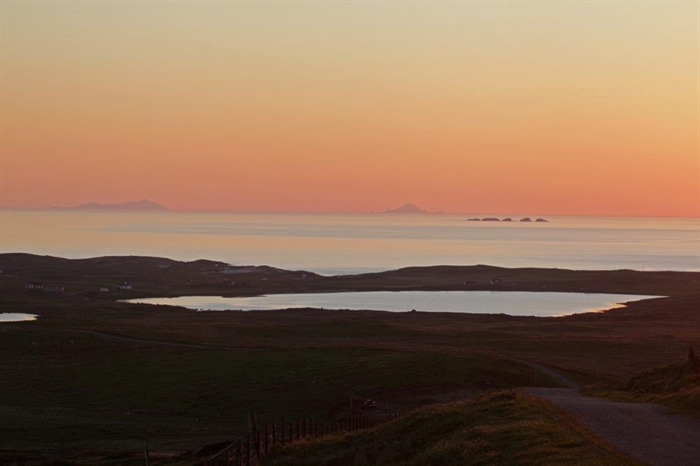The photograph captures a stunning canyon-like landscape at sunset. In the foreground, there is a darkened area with patches of grass and dirt, where a road curves from the bottom right and meanders up toward a cement pathway. A vehicle is faintly visible in the dirt at the bottom. As the scene extends into the background, a serene pond is revealed, leading up to a much larger, tranquil body of water, possibly an ocean or large lake. This expansive water feature is bordered by brownish terrain before fading into light gray silhouettes of distant hills. The sky above is a gradient of vibrant colors—pink at the lower horizon transitioning to yellow towards the top—reflecting the sun's setting rays and casting an orange and yellow glow over the entire landscape. The clear and detailed scenery underscores the natural beauty and tranquility of this outdoor vista.